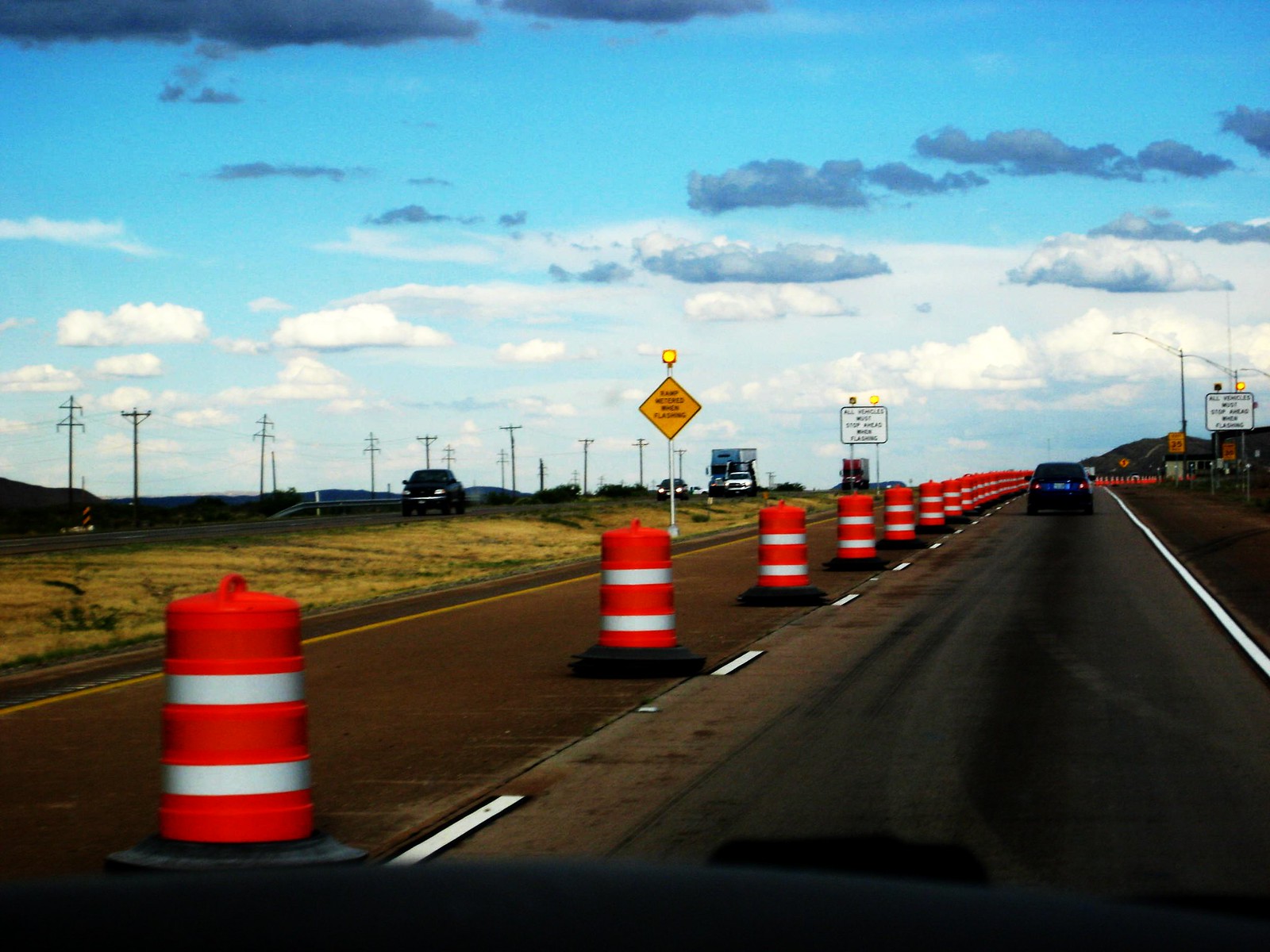This photograph captures a scenic moment from inside a vehicle traveling along a rural four-lane highway in the United States. The perspective places the viewer on the right-hand side of the highway, moving in a direction that features a substantial grassy median dividing the opposing lanes. Ahead of the vehicle, a car with its brake lights illuminated is evident, suggesting a potential slowdown due to the traffic conditions.

The sky above is a dramatic tapestry of various shades of blue, interspersed with white, light gray, and darker gray fluffy clouds, adding depth and mood to the scene. The roadway on this side is lined with a sequence of orange and white cylindrical barricades, which extend into the distance before veering to the right, indicating a possible lane closure or construction zone.

Across the median, a sparse number of vehicles, including several trucks and semi-trucks, cruise along in the opposite direction, underscoring the tranquility and lower traffic density typical of country highways. A small, yellow, diamond-shaped sign is partially visible, though its text is too diminutive and blurred to decipher clearly; it appears to include the word "flashing," possibly signaling a caution or construction notice.

Overall, the image captures a moment of rural travel under an expansive and variable sky, marked by subtle indicators of ongoing roadwork and vigilant driving.